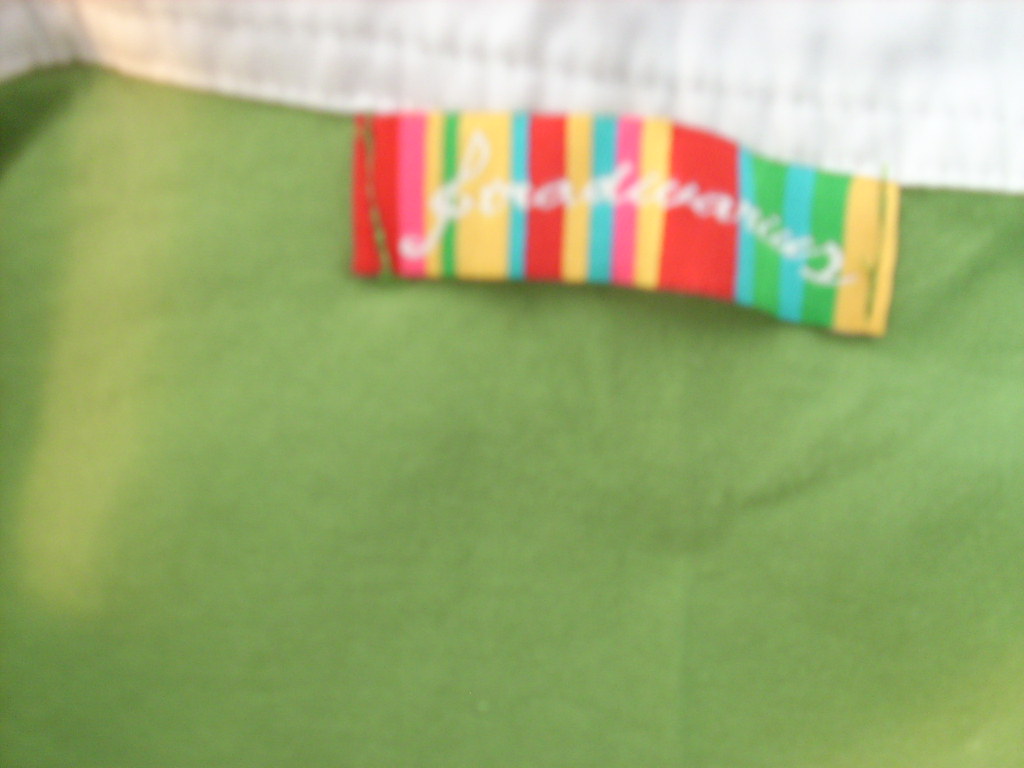The image is a very blurry and zoomed-in photograph, seemingly of an article of clothing, possibly a blanket or shirt, with a distinct tag prominently displayed. The main fabric appears to be green, potentially felt given the fuzzy appearance, suggesting a new and unworn item marked by visible seams. The top portion features a white or light violet trim that could be a collar or frock-like addition. The tag itself, which stands out due to its colorful vertical rainbow stripes, contains cursive writing that is indecipherable but flows elegantly across the label. The overall quality of the picture indicates it might have been cropped from a larger image, explaining its lack of clarity.